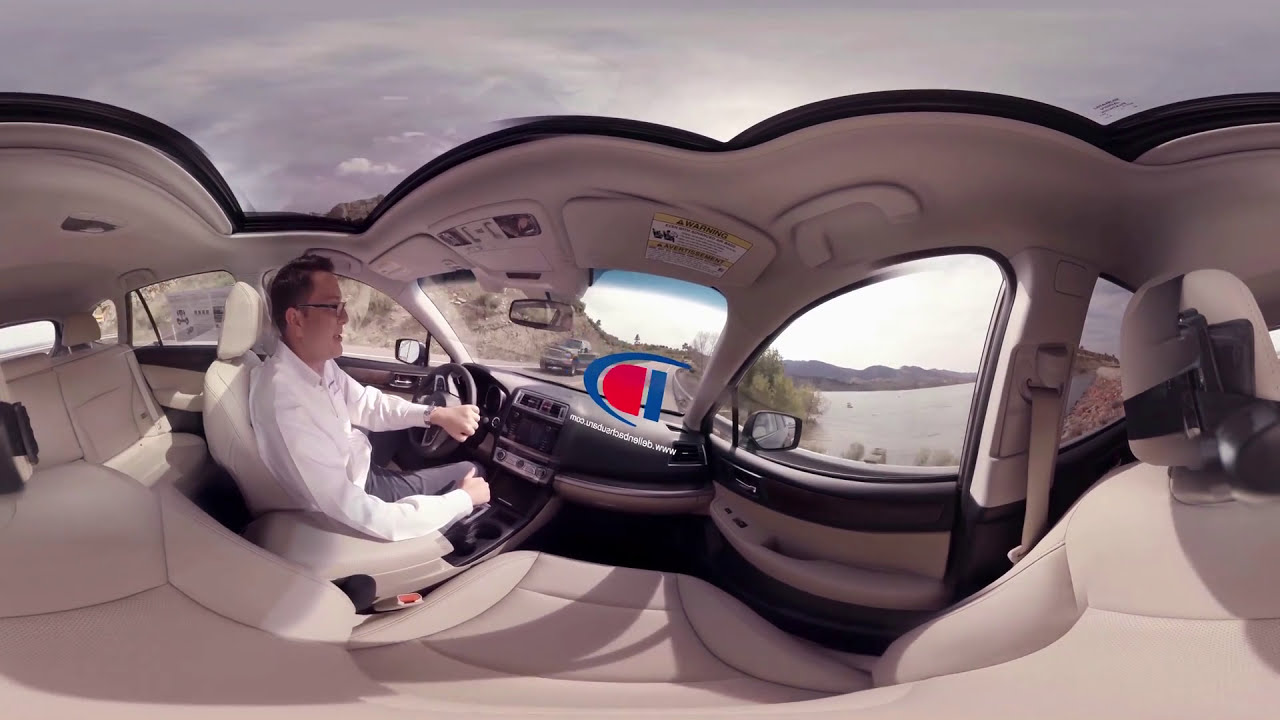A detailed 360-degree panoramic shot captures the interior of what appears to be an SUV, showcasing a man in a white long-sleeve dress shirt and black pants, possibly an older Asian gentleman wearing glasses, as he drives along a highway. The vehicle has a gray-ish upholstery with a beige roof and a black dashboard with beige accents. The image features noticeable distortions typical of a 360-degree shot. The driver is seen with his left hand on the steering wheel, seemingly turning right and possibly speaking, suggesting this might be a screenshot from a video, potentially designed for virtual reality. The panoramic camera, possibly taped to the passenger seat headrest, reveals a broad outside view. To the right, you see a large lake or river bordered by trees, vegetation, hills, and mountains in the background. On the left, there is a tall wall and some more trees, contributing to the rural setting. A distorted website address appears in the center of the image. Additionally, the windshield shows a red and blue sign, possibly for a business, and an oncoming black car is visible in the background. The ceiling might be clear, suggesting the possibility of the vehicle being a convertible.